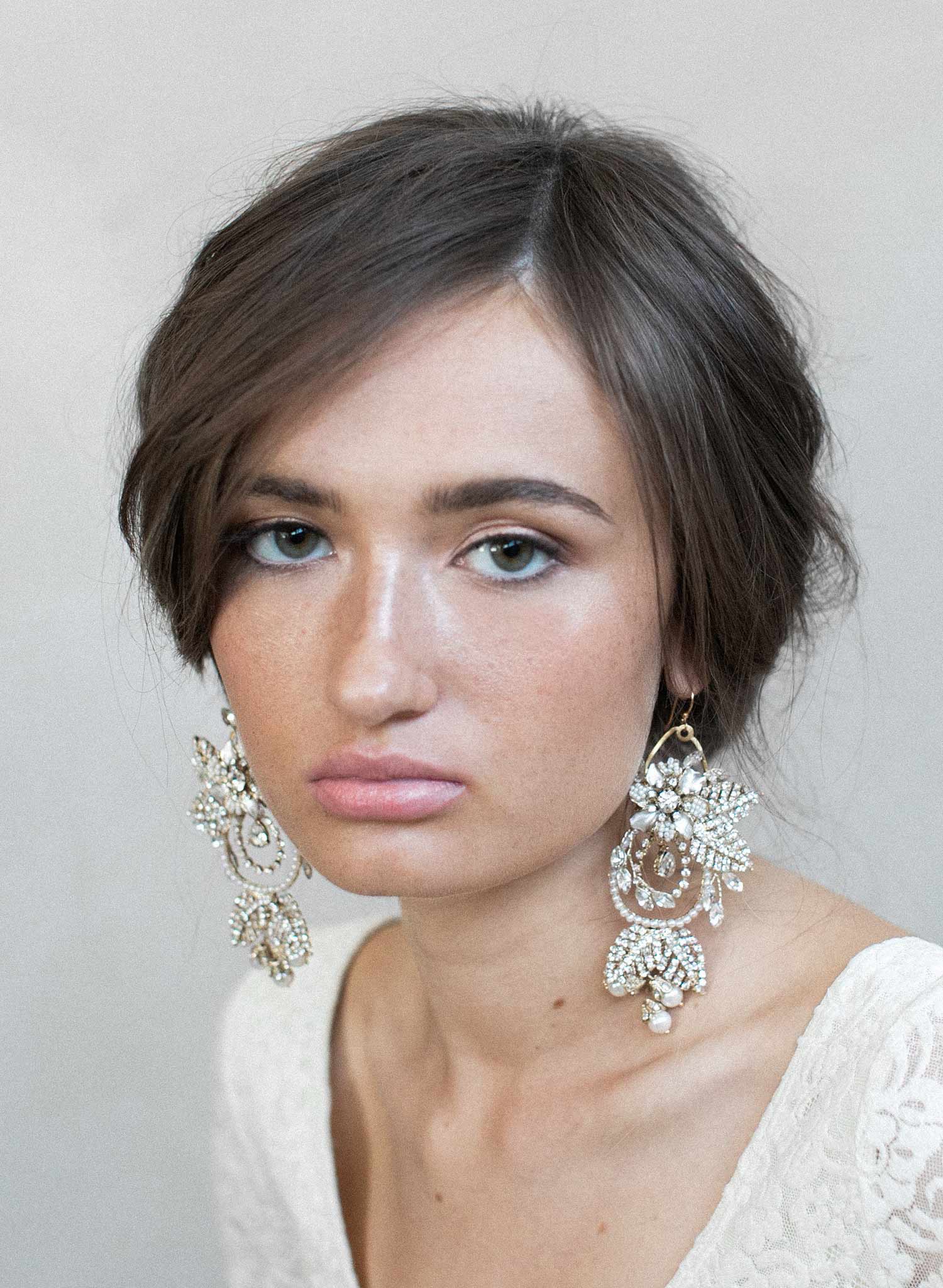The photograph captures a young woman in her late 20s with dark brown straight hair, pulled back, possibly into a ponytail or bun. Her slightly parted hair frames her face, which is marked by strong, dark eyebrows. Her greenish-brown or hazel eyes are deep-set and enhanced with slight brown eyeliner, dark mascara, and a subtle peach or tan eyeshadow. She wears natural makeup with light pink lipstick that highlights her arched brows. Her expression is notably unhappy or sad, with a gaze that feels direct and poignant.

She dons large, intricate earrings that dangle gracefully to her prominent collarbones. These earrings are florally designed with hoops and leaves, made from a white crystal material, possibly rhinestones. Her attire consists of a white top, which is low-cut with lace sleeves, perfectly complementing her olive-toned skin. The photograph is cropped just below her collarbones, ensuring a focused view of her upper body and face, capturing the depth and emotion in her expression, and the elegance of her appearance.